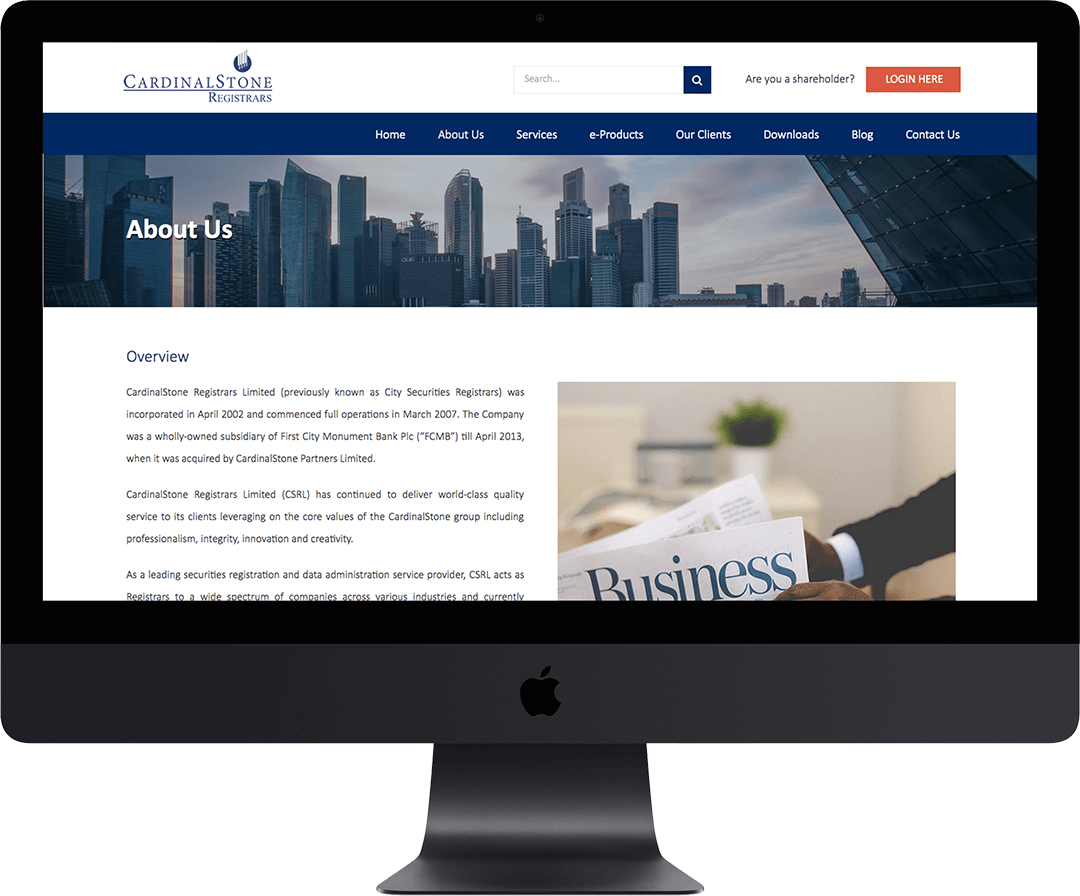An image shows a sleek Mac desktop characterized by its dark gray base and border, centered around a black Apple logo. The screen displays the homepage of a website called "Cardinal Stone." In the top-left corner of the page, the text "CARDINAL STONE" features substantial character spacing and is colored blue. Beneath this header, towards the right, a blue line divider precedes the word "Registrars." An eye-catching circular blue icon, depicting several white books, overlays the Cardinal Stone logo.

The website's interface includes a menu bar with a dark blue background. Starting from the center and moving rightwards, various menu options in a basic white font are listed sequentially: Home, About Us, Services, e-P, Products, Our Clients, Downloads, Blogs, and Contact Us. Below this menu bar is a banner showcasing several white and gray corporate buildings set against a cloudy sky backdrop. Overlaying the left side of this banner is the white text "About Us."

The next section of the webpage transitions to a white background, displaying the word "Overview" in black. This section contains around two and a half paragraphs of small black text outlining the business's details. Additionally, there is a stock photo featuring a setting with white walls, a white pot holding a green plant in the background, and two hands in black suits with white undershirts holding a newspaper titled "Business."